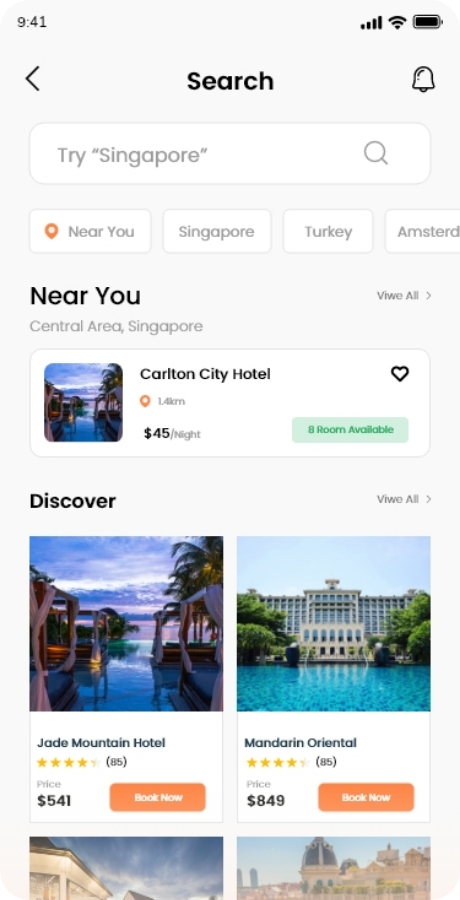This image captures a screenshot of search results on a mobile phone, timestamped at 9:41. The top of the screen displays standard mobile status icons, including Wi-Fi, battery, and network signals. Positioned beneath is a row that features a search icon on the left, a greater-than symbol, and a bell or alert icon on the far right.

Centered on the page is a search bar with the query "Try Singapore". Directly below, there are four suggestion boxes labeled: "Near You," "Singapore," "Turkey," and "Amsterdam". Beneath these, the heading "Near You" appears, with an option to "View All".

Currently shown under the "Near You" category is "Carroll City Hotel," which offers rooms at $45 per night and has eight available rooms. Following this is a bold "Discover" section listing two prominent hotels: "Jade Mountain Hotel" at $541 per night and the "Mandarin Oriental Hotel" at $849 per night. There are two additional clipped photos of hotels that are partially visible without names or prices.